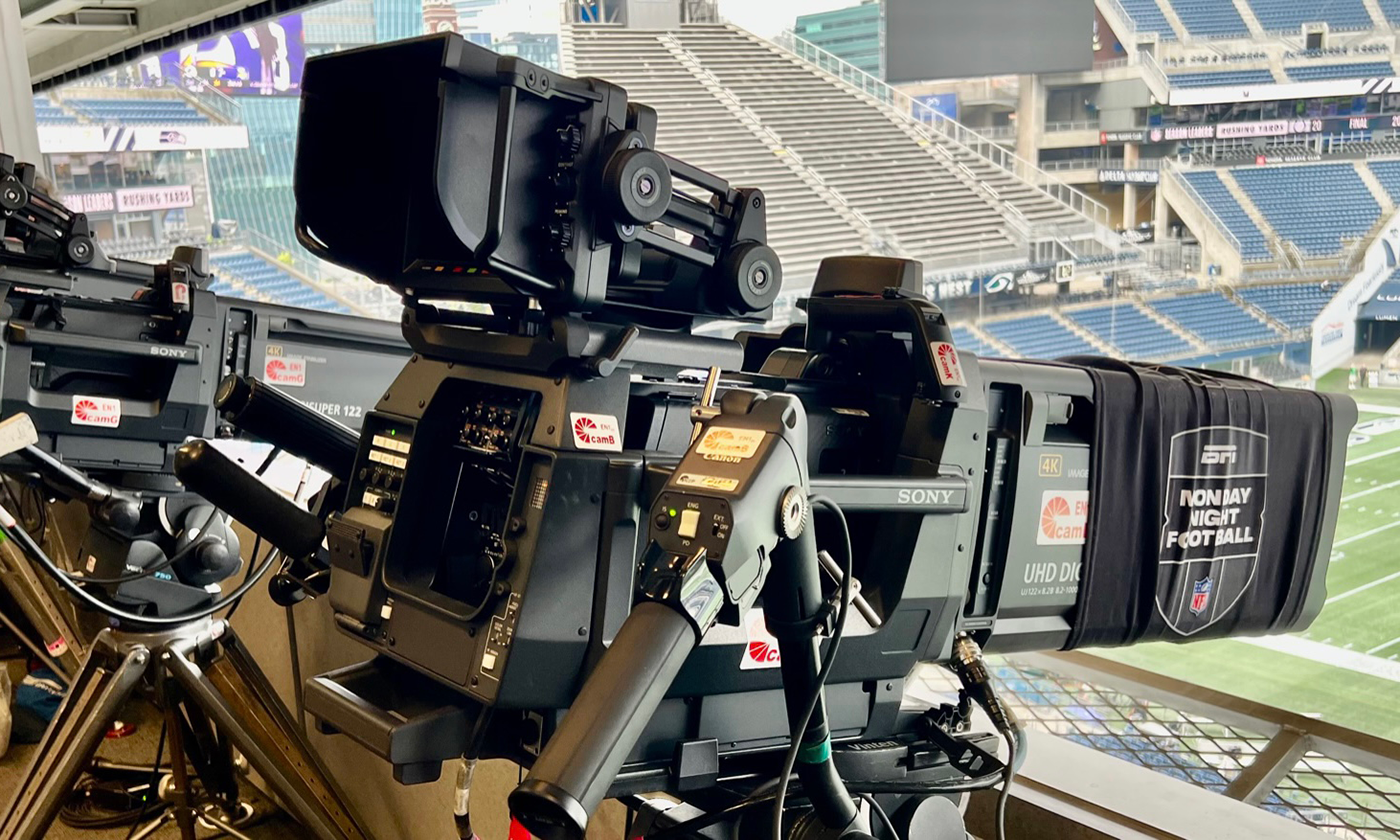The photograph is a full-color, horizontally rectangular image taken indoors, although the light source is ambiguous. The primary focus is on a pair of unmanned, black TV cameras, prominently displaying several white labels with red text. Each camera features numerous intricate controls, levers, and handles, highlighting their complex design. 

Wrapped around the lens hood of the foreground camera is a black cloth emblazoned with the ESPN Monday Night Football logo in large, white, uppercase letters, along with the NFL logo below it. This cloth adds a distinctive touch and indicates the cameras' purpose. The side of the camera also bears the "Sony" logo in white. 

In the background, the setting reveals an empty outdoor football stadium. The upper left corner of the image shows blue and gray but empty stands, with visible stripes of the American football field towards the lower right. A second camera, similar in design, is situated slightly behind and to the left of the primary camera, but it's less prominent in the composition. The scene is devoid of any personnel, contributing to a serene and undisturbed atmosphere.